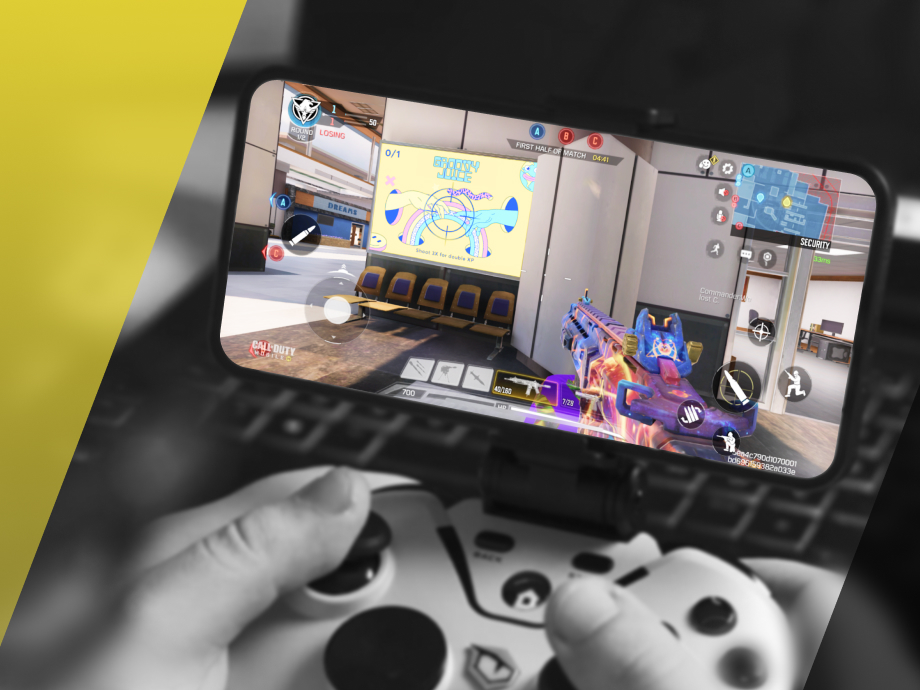This image features a visually striking blend of black and white and color elements. The main portion of the photo is in black and white, drawing immediate attention to the brightly colored elements. Set against a vivid yellow backdrop, a child's hands are seen gripping a joystick video game controller with an eye-shaped logo on the center button. Attached to the controller is a smartphone in a horizontal position, acting as a display for a vibrant first-person shooter game. 

In sharp contrast to the monochrome surroundings, the game screen is exceptionally colorful, with hues of purple, pink, blue, and yellow dominating the scene. The player's perspective shows a gun in a kaleidoscope of colors, aiming towards a sign emblazoned with blue text reading "spoofy juice," flanked by two hands pointing at each other, reminiscent of classical art styles. Above the sign, a rainbow arches gracefully in shades of blue, purple, yellow, and pink, and an intriguing "0/1" counter is displayed in gray text.

The game interface includes various control icons: bullets, a man kneeling, and a directional control circle for navigation, suggesting this might be a first-person shooter game. In the top right corner, a minimap with colored dots — red, blue, and yellow — marks key locations or objectives.

In the background of the game screen, an indoor scene unfolds with rows of chairs featuring purple cushions and a billboard in pale yellow, blue, and light green. There’s also an office space with a desk and computer screen visible on the right side of the game display. Underneath the smartphone, a keyboard is faintly visible, indicating the presence of a laptop possibly on the child's lap, completing this highly detailed and dynamic snapshot of modern handheld gaming.